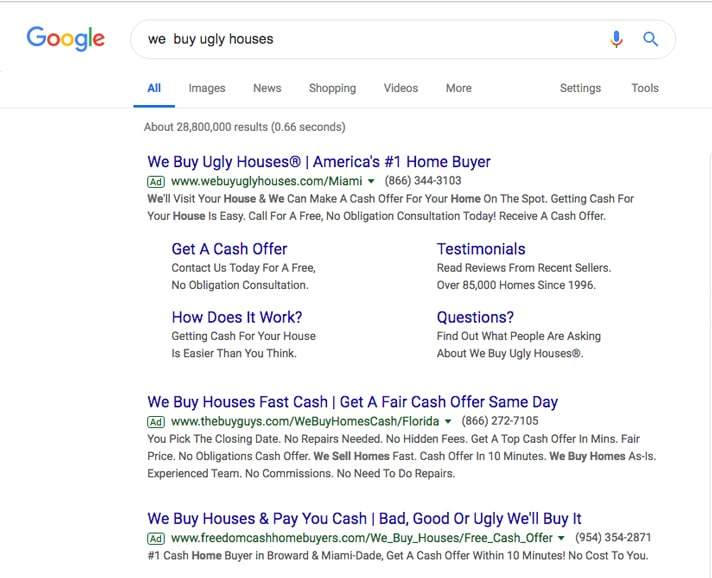The image depicts a Google search results page. Prominently displayed in the top left corner is the Google logo, rendered in its signature colors: blue, red, yellow, blue, green, and red. Below the logo is the search bar with the query "we buy ugly houses" typed into it. Just beneath the search bar, categories for results appear, including "All," "Images," "News," "Shopping," "Videos," "More," "Settings," and "Tools."

The search results indicate approximately 28,800,000 results in 0.66 seconds. The first result appears to be an advertisement for a company branded as "We Buy Ugly Houses®," described as America's number one home buyer. The advertisement details the company's promise to visit homes and make cash offers on the spot, emphasizing the ease of the process by highlighting a free, no-obligation consultation. It stresses the advantages of receiving a cash offer quickly, regardless of the condition of the house—be it bad, good, or ugly.

Additionally, the ad mentions various sections such as "Testimonials," "How does it work?" and "Questions," designed to provide more information to potential sellers. The background of the Google page is predominantly white, and familiar UI elements like the magnifying glass search icon and the voice search icon are present. The color scheme used on the page aligns with Google's classic blue, green, red, and yellow palette.